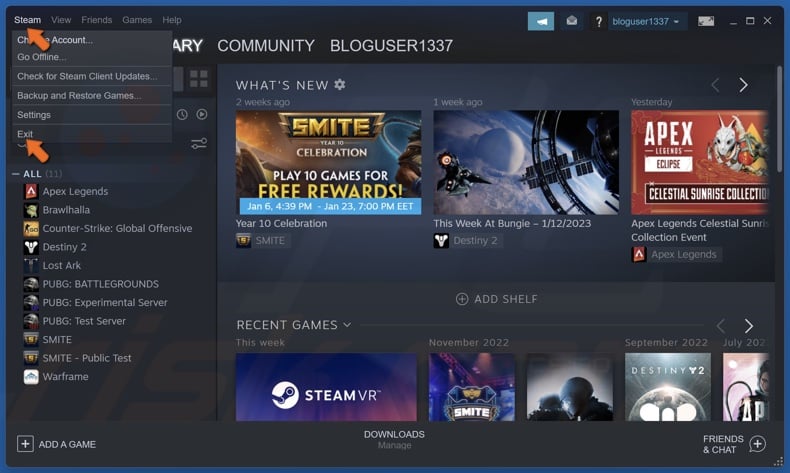**Detailed Caption:**

This screenshot depicts a user's interface on the Steam platform, characterized by a dark grey background prevalent throughout the image. Prominently displayed at the top left of the screen are the following menu options: *Steam, Create Account, Go Online, Check for Steam Client Updates, Backup and Restore Games, Settings,* and *Exit*. Two orange arrows draw attention to the *Steam* dropdown menu, while another points to the *Exit* option.

Beneath this menu, a vertical list showcases several game titles under the heading beginning with *All*, followed by *Apex Legends, Brawlhalla, Counter-Strike: Global Offensive, Destiny 2, Lost Ark, PUBG Battlegrounds, PUBG Experimental Server, PUBG Test Server, SMITE, SMITE Public Test, Warframe,* and concludes with an *Add a Game* option.

Dominating the main area of the screen, there are various sections such as *Community, Blog User 1337,* and *What's New*. Featured prominently are various promotional banners and game listings: *SMITE Celebration, Play 10 Games for Free Rewards, This Week at Bungie* (dated 1-12-23), *Apex Legends Eclipse,* and *Celestial Sunrise Collection*. 

Towards the bottom of the main screen, a segmented section includes an *Add Shelf* option, followed by *Recent Games* and *SteamVR*. Listed underneath are several game titles including *November 2022, SMITE, Destiny 2*, with another game partially cut off from view.